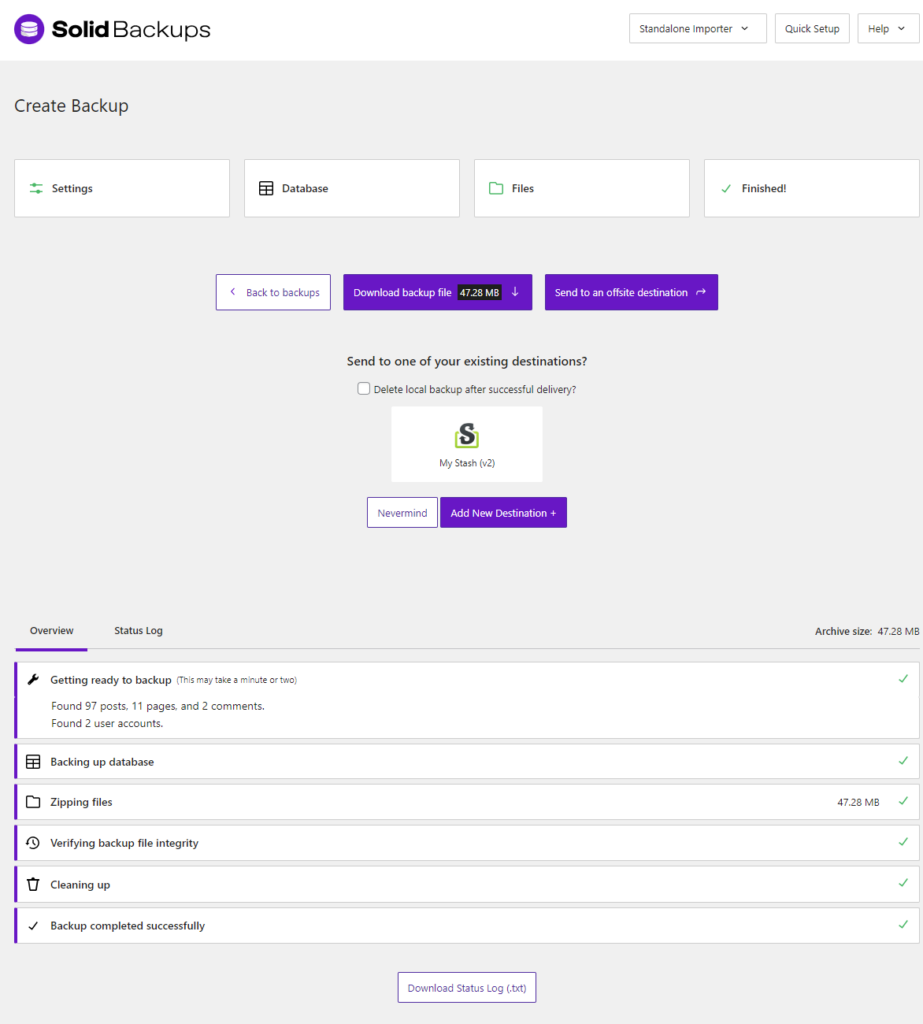Screenshot of a web page showcasing the "Solid Backups" software interface:

- **Top Section:**
  - **Top Left Corner:** "Solid Backups" logo or text.
  - **Top Right Corner:**
    - Three gray buttons:
      - "Stand Alone and Porter" with a downward arrow for a dropdown menu.
      - "Quick Setup."
      - "Help" with a downward arrow for additional options.

- **Sidebar (Left Side):**
  - Gray button labeled "Create Backup."
  - Below that, a series of white rectangular buttons:
    - "Settings."
    - "Database."
    - "Files."
    - "Finished."

- **Middle Section:**
  - Midway down the left side, a gray text with a right-facing arrow: "Back to Backups."
  - Center and middle-right section features two prominent purple buttons:
    - "Download Backup File."
    - "Send to an Office Destination."

- **Lower Middle Section:**
  - Instruction in black text: "Send to One of Your Existing Destinations."
  - Unchecked checkbox with the label: "Delete Local Backup After Successful Delivery."
  - A white rectangle containing:
    - A large black "S" with a green square.
    - The text "My Stash W2."
  - Lower down, two buttons:
    - "Nevermind."
    - "Add New Destination."